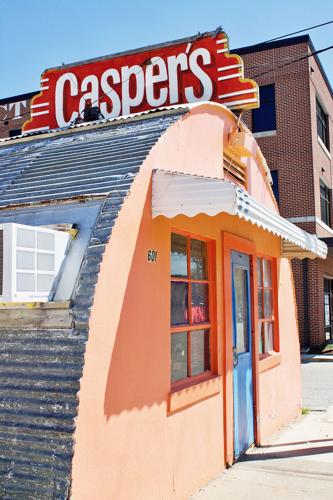The image depicts a small, roadside diner styled after an old military barrack or airplane hangar, characterized by its distinctive half-circle, cylindrical shape. The building features peach-colored, corrugated steel siding with horizontal ridges, and a white metal roof. On the left side, a white in-window air conditioning unit is visibly installed. The front of the diner is marked by a blue door with a large rectangular window occupying its upper half. Flanking the door are two grid-style windows, one on each side. A simple, white metal awning extends over the entrance. Above, a prominent red sign with curvy sides and yellow trim displays "Casper's" in large white letters, possibly in a retro 1950s-style font. Behind the diner, a three to four-story brick building and a network of power lines are set against a clear blue sky. Along the ground level, there is a concrete sidewalk completing the scene.